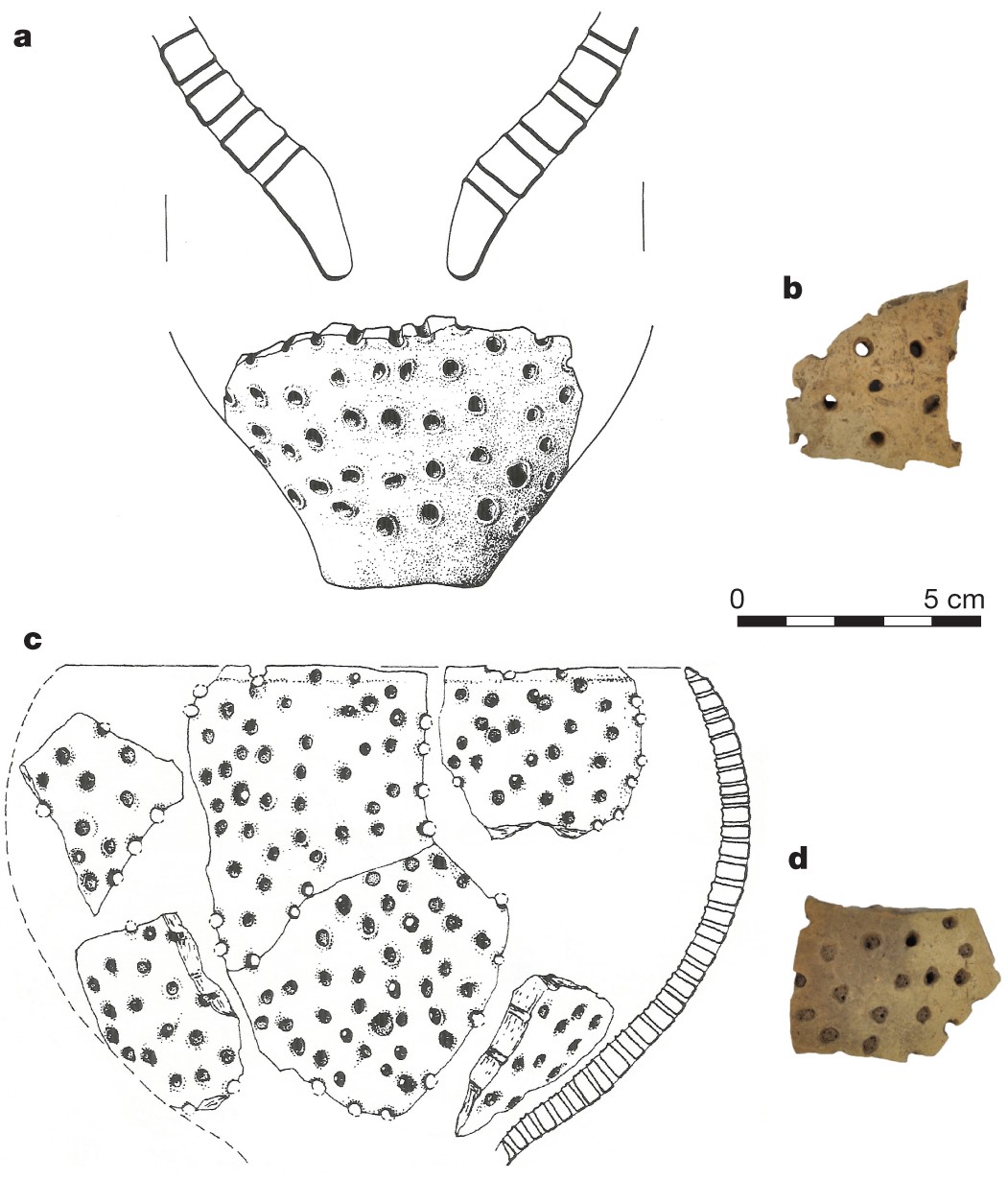The image is a detailed diagram featuring four sections labeled A, B, C, and D. At the top left corner, labeled 'A,' is a black-and-white drawing showcasing bone-like structures with circular holes, reminiscent of a rock or hard material. Hanging from this section are two snake heads. Below 'A' is 'C,' another black-and-white illustration similar to the first, with more pieces of the hole-riddled material arranged in a squarish pattern. To the right of 'A,' labeled 'B,' is a brown, real-world photo displaying a piece of pottery with numerous holes, seemingly broken off from a larger, rounded artifact. Correspondingly, 'D' at the bottom right mirrors 'B' with another photo of a similarly holed pottery fragment, suggesting reconstruction from historical or archaeological findings. Overall, the diagram contrasts artistic renderings on the left with actual photographic evidence on the right, emphasizing the reconstruction of these perforated artifacts.